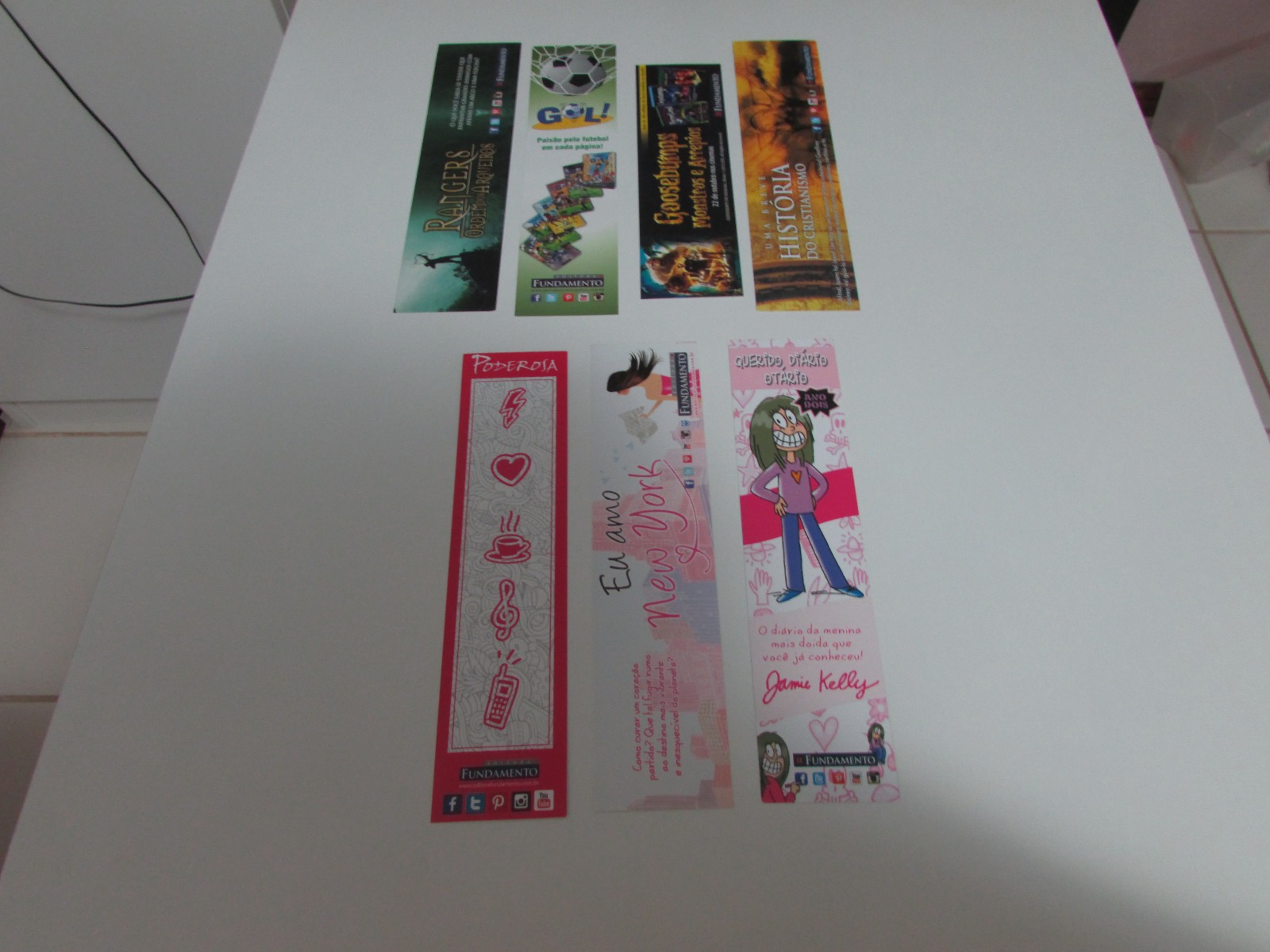This angled photo taken indoors showcases seven rectangular bookmarks arranged on a pristine white table. Each bookmark is distinct, exuding a youthful appeal through an array of vibrant hues such as pinks, blues, and greens. These bookmarks serve as promotional tools, each hinting at a different theme or series: one advertises the 'Goosebumps' series, another displays historical content with "History" written on it, while others feature various symbols, photos, and playful cartoons. Notably, one bookmark prominently features a pink border adorned with drawings of a coffee cup, musical note, heart, lightning bolt, and a mobile phone, all in pink. Social media icons for platforms like Facebook, Twitter, Pinterest, and Instagram are stamped uniformly across all bookmarks. The background details include a white wall with visible black wires in the top left and a white floor with dirty grout in the top right corner, adding a subtle, lived-in feel to the scene.